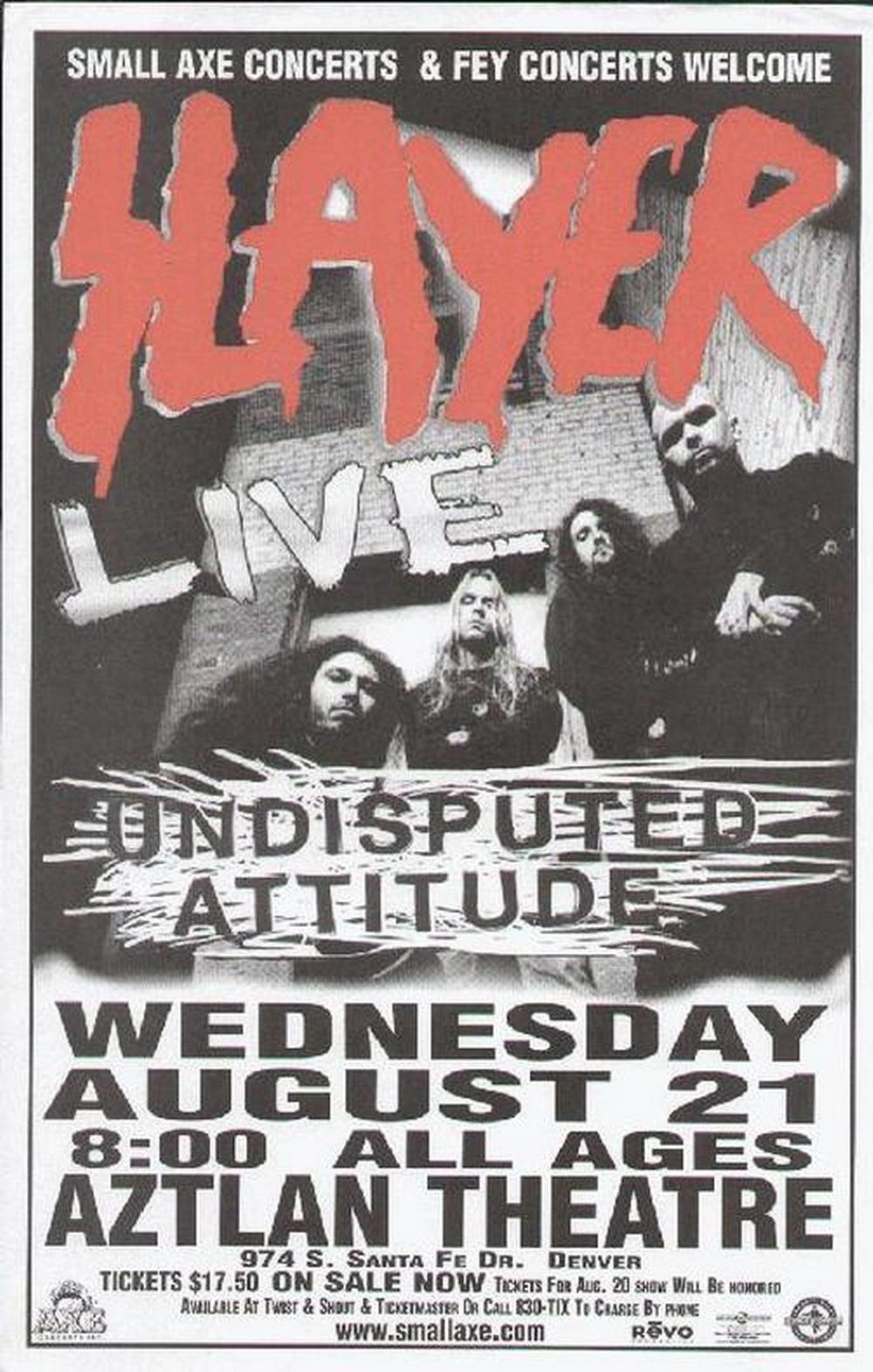The concert poster is a monochromatic black and white design with striking red text at the very top that reads "Slayer" in their iconic logo style. The poster announces "Small Axe Concerts and F.E.Y. Concerts Welcome Slayer" in white text above the band's name. Below Slayer's red logo, it states "Live" in white text and "Undisputed Attitude" in black text with a white scribbled background.

Centered on the poster, there's a black and white photograph of Slayer's four members standing outside a brick building. The band's lineup includes a mix of long-haired and bald members, all dressed in black. The image perspective is slightly angled upwards as if taken from the ground, giving the band a towering presence.

Details about the concert follow beneath the photo. The event is scheduled for Wednesday, August 21st at 8 PM, held at the Astland Theater located at 974 South Santa Fe Drive in Denver. The concert is open to all ages, with tickets priced at $17.50. Tickets are available for purchase now at local shops like Twist and Shout, with phone orders also accepted. Finally, the bottom of the poster features various sponsor logos and the website smallaxe.com for additional information.